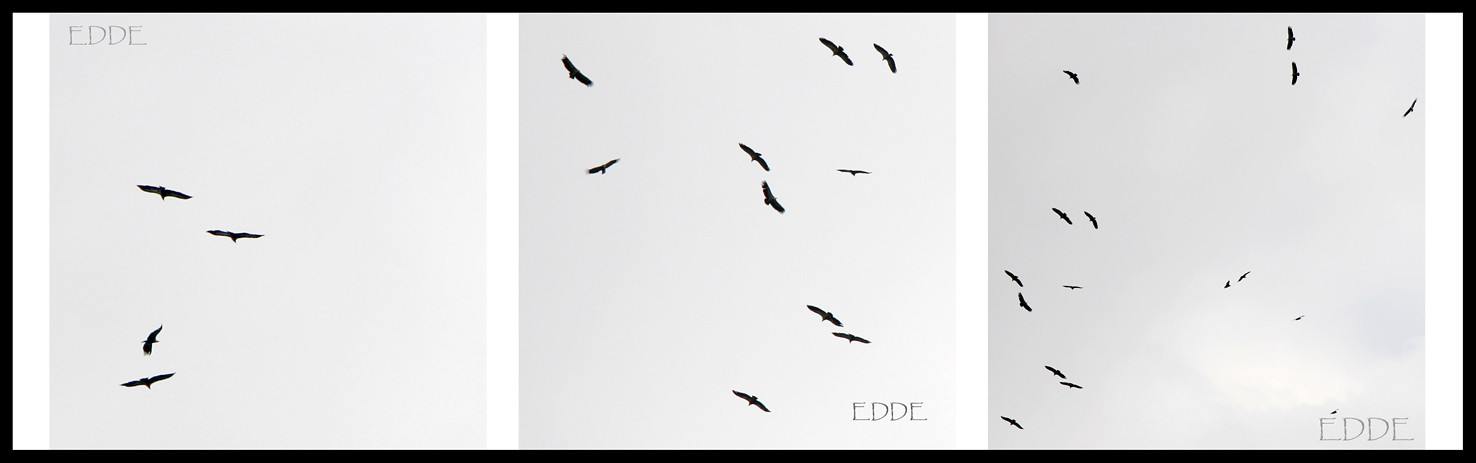This color photograph features a triptych framed by a black outline, each of the three inner pictures having a subtle pink overlay. The images, designed in shades of gray that progressively darken from left to right, depict birds—likely crows or seagulls—in mid-flight against a sky. Each section of the triptych bears the letters "E D D E" in all capital letters; the first set of letters appears at the top of the leftmost frame, while the bottom two sets are at the bottom of the middle and rightmost frames. In the first frame, there are four birds crisply captured. The middle frame shows around ten birds, and the final frame features numerous birds that appear smaller and are flying farther away.